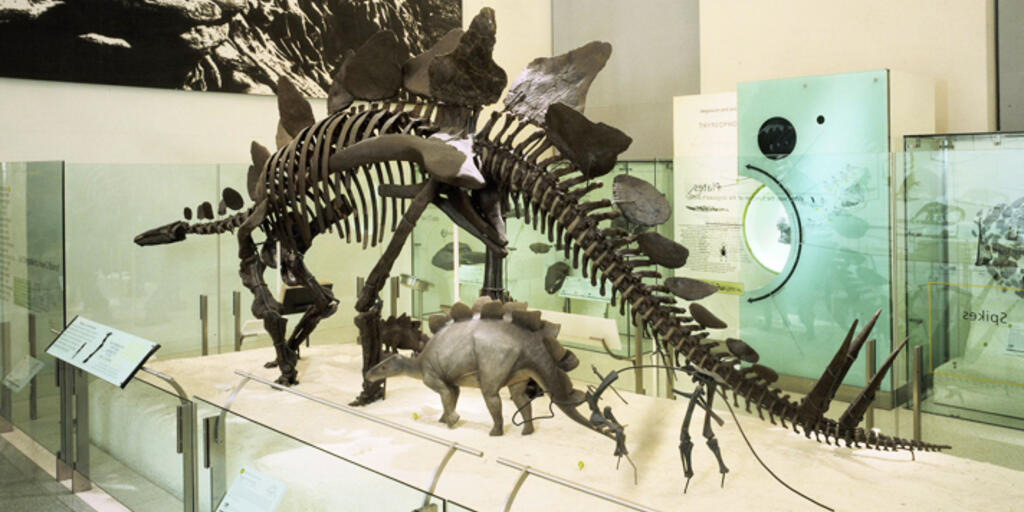The photograph showcases a detailed display within a history or science museum, prominently featuring the large skeleton of a Stegosaurus. The skeleton, which appears dark brown in color, is mounted on a pristine white display platform that also includes a stark white placard, though the text on it remains illegible from the photograph's angle. Directly below the towering skeleton is a small, photorealistic model of a full-bodied Stegosaurus, providing a visual representation of the dinosaur in lifelike detail. The scene is encased with glass dividers, emphasizing the importance and preservation of the exhibit. In the background, slightly blurred but visible, are various poster boards or depictions related to the exhibit, adorning the wall behind the display. This setup suggests a typical, well-curated museum exhibit likely to attract tourists and educational enthusiasts.